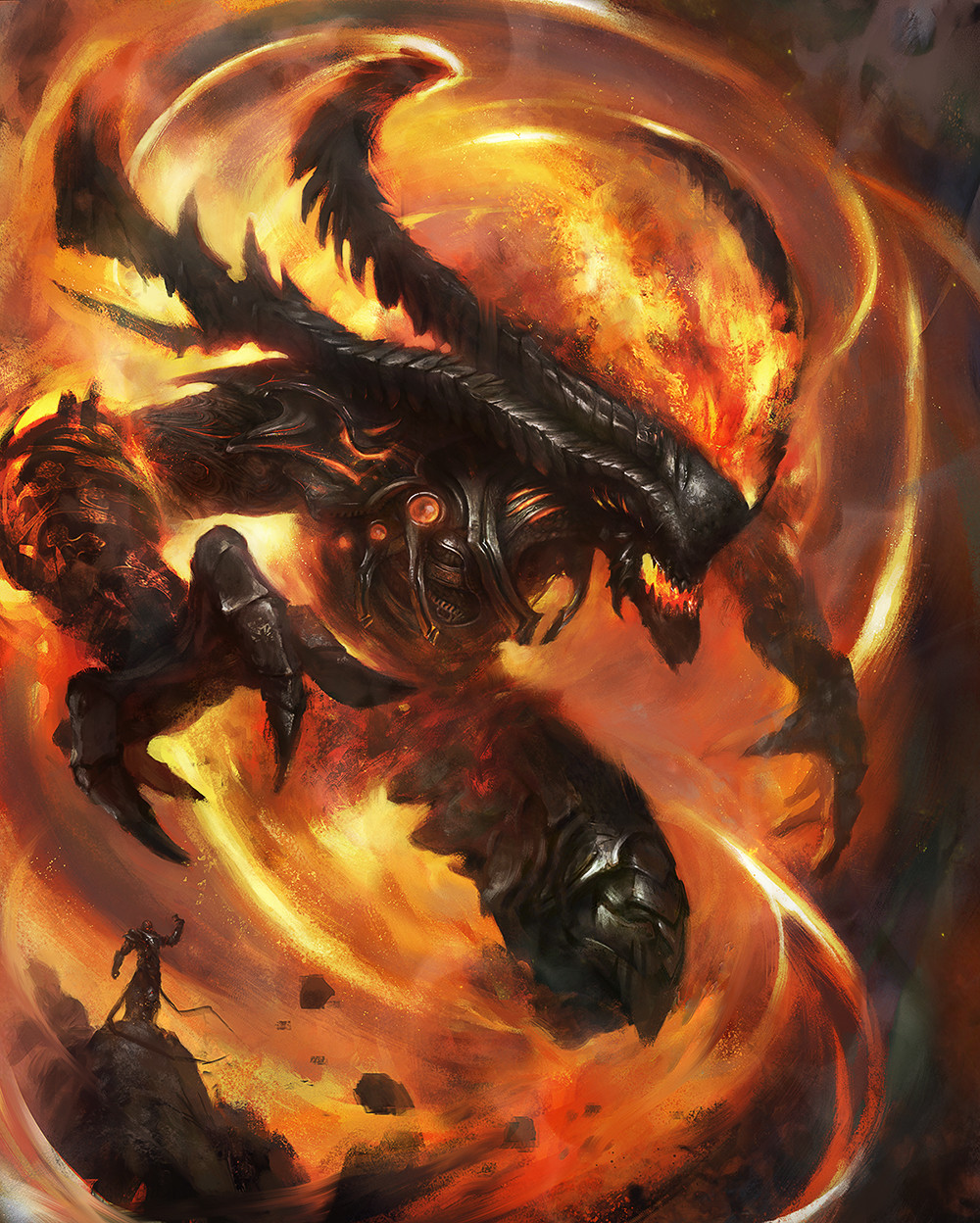The image is a highly detailed, fantastical color drawing depicting a terrifying, metallic monster emerging from a fiery abyss. The creature, reminiscent of a blend between a dragon, a bug, and an alien from the Ripley films, projects a menacing aura with its sharp, jagged mouth and prominent claws. The alien-like monster appears as if it's coming through from another dimension, engulfed in swirling orange and black flames that illuminate its glowing orange eyes. The background is ablaze with fiery swirls, creating a hellish landscape reminiscent of Dante's Inferno. In the lower-left corner, a much smaller, human-like figure stands on a rocky outcrop, clad in metallic garb with extended limbs. This figure, with one arm raised in a summoning gesture, adds to the scene's drama, as if orchestrating the emergence of this fearsome beast from the fire. The overall composition exudes a sense of impending danger and otherworldly power.